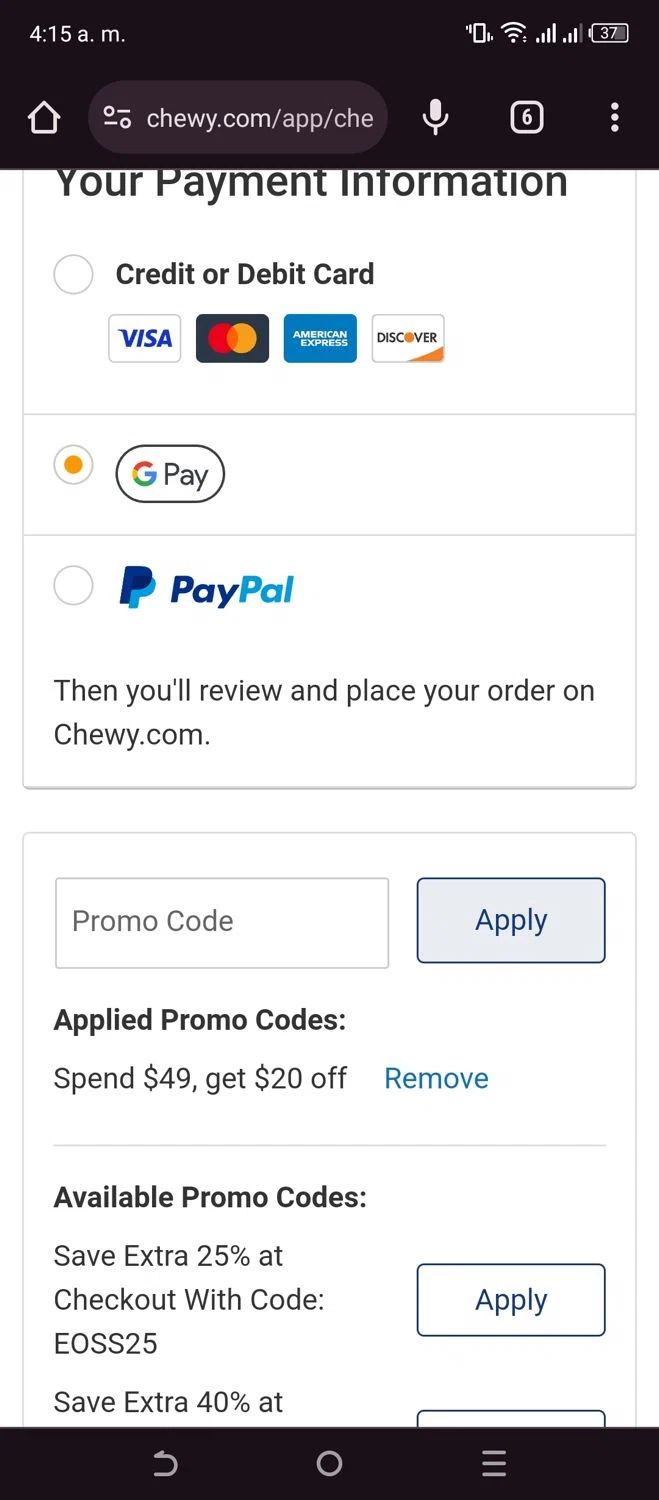This image displays a screenshot from a mobile device, showcasing the payment and promotional code section of a checkout page on Chewy.com. At the top, the URL "Chewy.com/app/che" is partially visible, cut off mid-text. The heading "Your Payment Information" is prominently displayed, indicating various payment options available to the user.

Presented below this heading are icons for accepted cards, including Visa, Mastercard, Discover, and American Express. Additionally, the screenshot highlights the selection for Google Pay, marked by a circular button filled with an orange dot, indicating it has been chosen.

Adjacent to these payment options is a blank section for PayPal, suggesting the user has not selected this method. 

Further down the page, there is instruction to "Review and place your order on Chewy.com," followed by an area reserved for entering promotional codes. This section includes a rectangular field labeled "Promo Code" with an adjacent blue "Apply" button.

Currently applied to the order is a promotional code offering "$20 off a purchase of $49 or more," which can be removed by clicking a provided button. Additional available promotions are also listed, such as a code for "25% off at checkout," with an option to apply this discount as well.